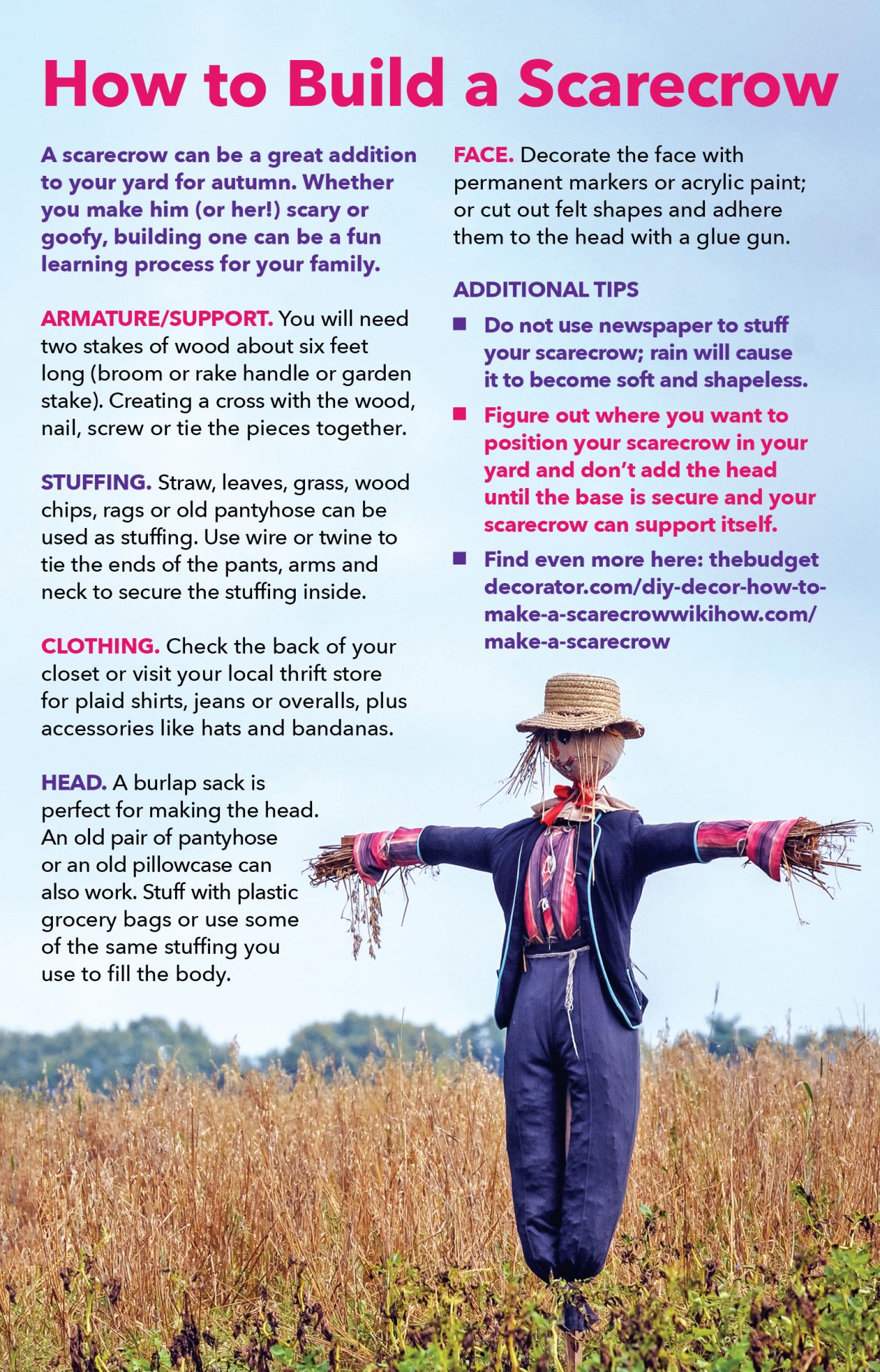The image features a vibrant informational poster titled "How to Build a Scarecrow" in bold fuchsia letters at the top. The poster is divided into several sections, detailed with helpful instructions on constructing a scarecrow, including the armature support, stuffing, clothing, head, and face. Additional tips are provided: avoid using newspaper for stuffing as it turns soft and shapeless upon getting wet, secure the base before adding the head, and position your scarecrow thoughtfully in your yard. The poster includes a link to additional resources: "thebudgetdecorator.com/DIY-decor-how-to-make-a-scarecrow" and "wikihow.com/make-a-scarecrow."

In the lower right corner, the image depicts a close-up of a scarecrow standing in a field of tall, brown grain with a backdrop of green trees and a bright blue sky. The scarecrow is dressed in a blue sweater layered over a blue and red shirt, along with blue pants, and is topped off with a straw hat. Various text colors, including pink, purple, and black, emphasize different sections on the poster, making it both informative and visually engaging.